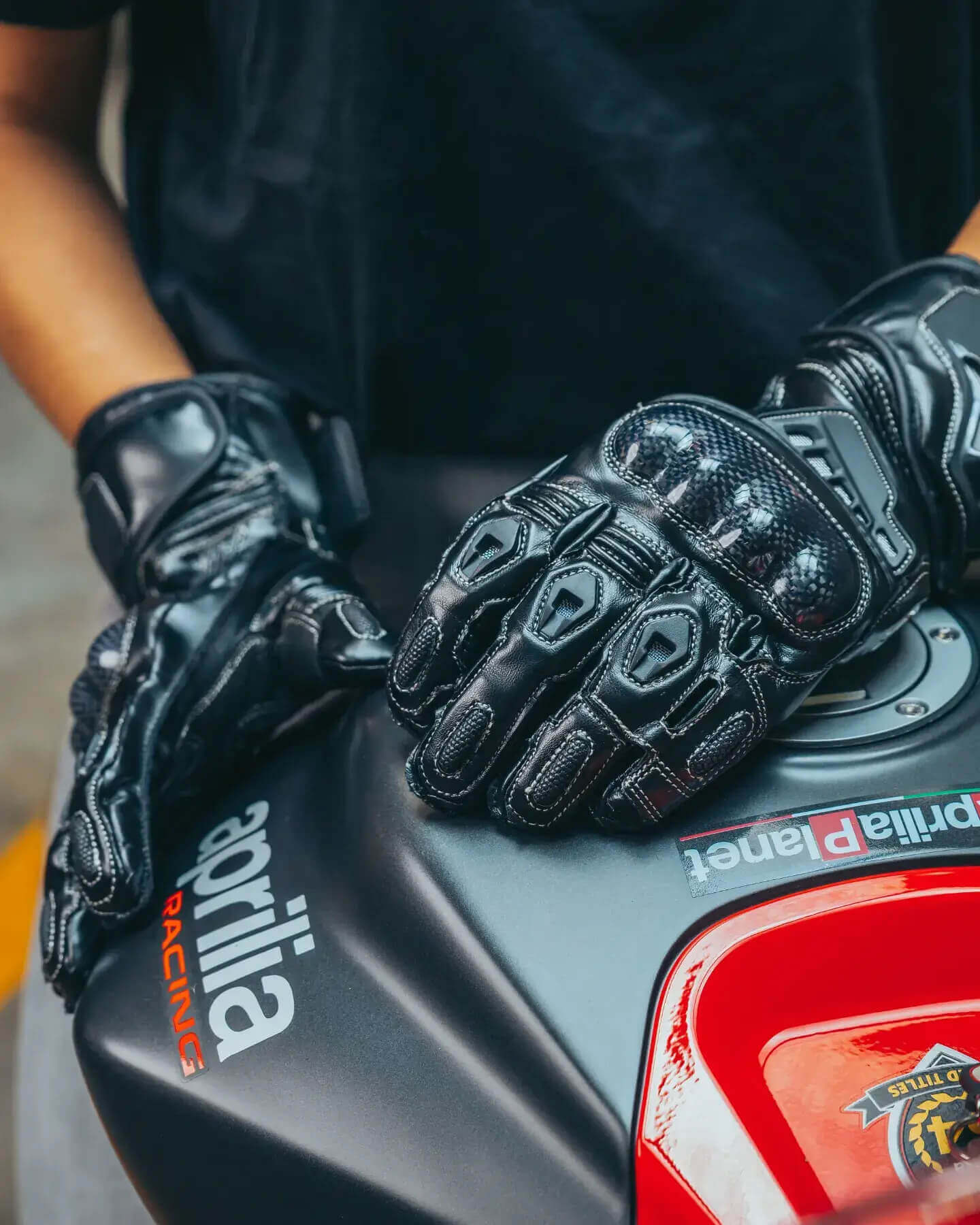This vertical, rectangular image captures a close-up view of a person from the chest down, showcasing their hands resting on a dark gray motorcycle tank adorned with labels, prominently featuring "Aprilia Racing" in orange capital letters. The individual is wearing a short-sleeved, dark blue t-shirt, revealing tanned, bronze-colored arms. The gloves they're wearing are high-quality, dark blue racing gloves that extend slightly past the wrist, equipped with dark blue Velcro straps for a snug fit. These gloves feature slightly lighter blue, shiny patches just below the fingers, and reinforced, honeycomb-patterned padding—possibly carbon fiber—on the knuckles for added protection. The overall look suggests these gloves are designed for serious motorcycle racing.